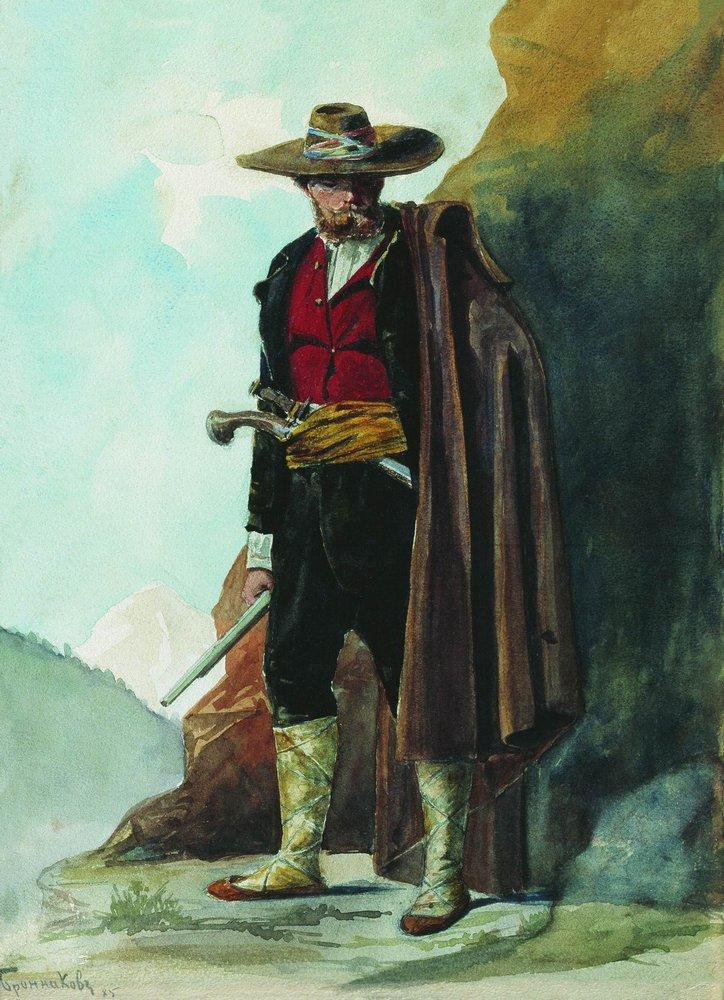The image depicts a finely detailed drawing of a stern and rugged Western man, exuding an air of toughness from an older time, perhaps the 1700s or 1800s, reminiscent of a cowboy or a figure from Spain or Mexico. Central to the image, the man stands with a wide-brimmed, circular sombrero adorned with decorations, casting a shadow over his eyes. His attire is elaborate: a white shirt beneath a red down-filled vest, topped with a golden-colored sash around his waist. Over his shoulder is a brown leather cape, and he wears black pants that reach just below his knee, tucked into tall white boots stained with green, white, and brown, suggesting an verdant terrain. In his right hand, he grips an old-fashioned rifle, with the barrel visible, while the hilt of another gun and possibly a knife or sword are tucked into his sash. His left hand is hidden beneath his cape. The background features a scenic landscape with distant mountains, blue sky with a few clouds, and some green grass near his feet, indicating a rugged yet picturesque setting. This piece, likely worthy of a museum, captures the essence of an era long past, portraying a figure you wouldn't want to cross paths with in olden days.